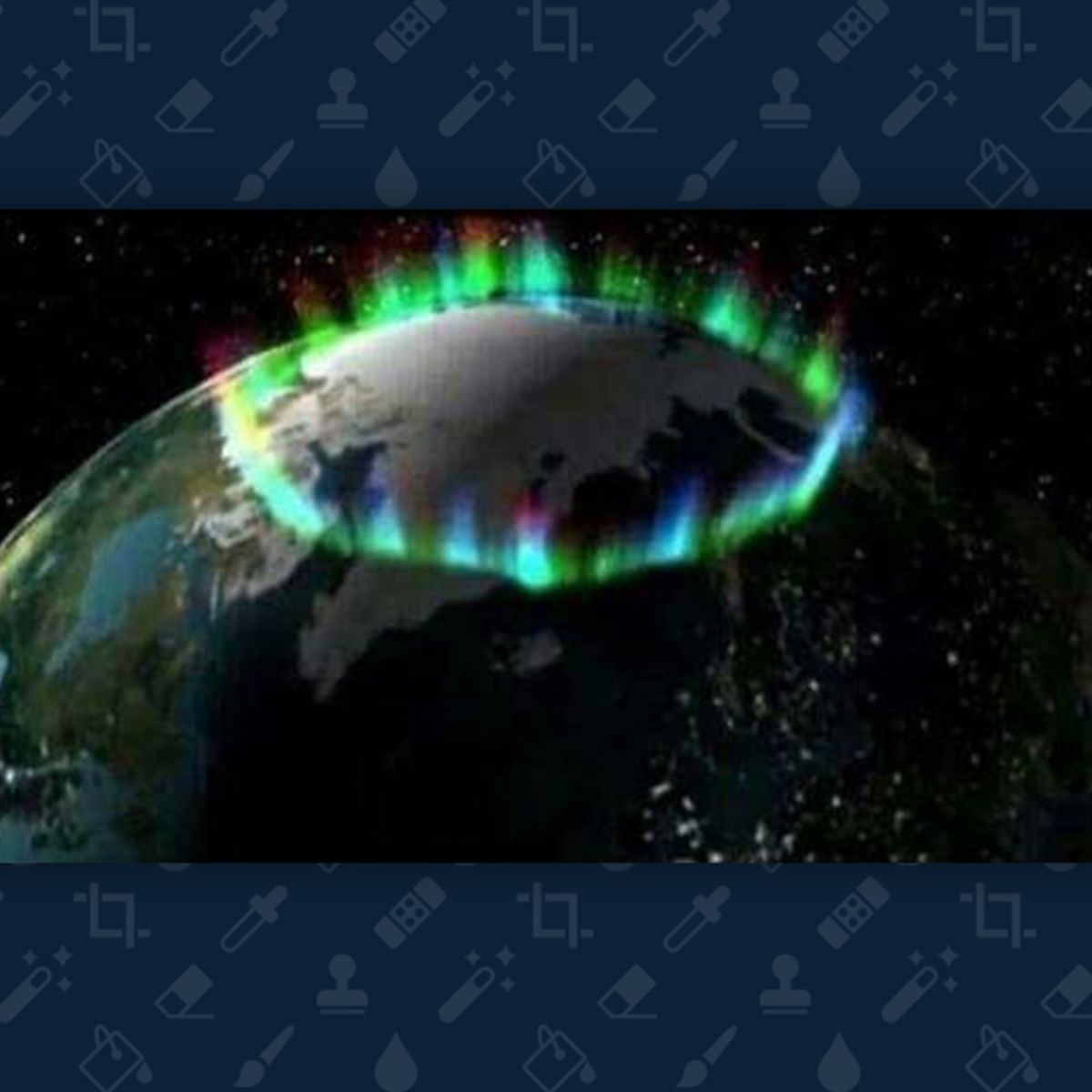The image presents a breathtaking perspective from space, showcasing the northern lights enveloping the entire top of Earth, resembling a luminous crown. The view appears centered over the Arctic region, potentially including parts of Asia and North America, lighting up the northern hemisphere with a spectacular display of predominantly green auroras, intertwined with hues of blue, pink, purple, and occasional bursts of yellow. The scene takes place against a dark backdrop sprinkled with white dots representing stars, emphasizing the cosmic setting. The border of the image is notable, adorned with a repeating pattern of scientific icons such as a crop signal, paintbrush, water droplet, and other objects, all working within a graphic design that adds an informative yet artistic frame to the visual feast. Despite some pixelation, the ethereal beauty of the auroras and the grandeur of this celestial event are vividly palpable.